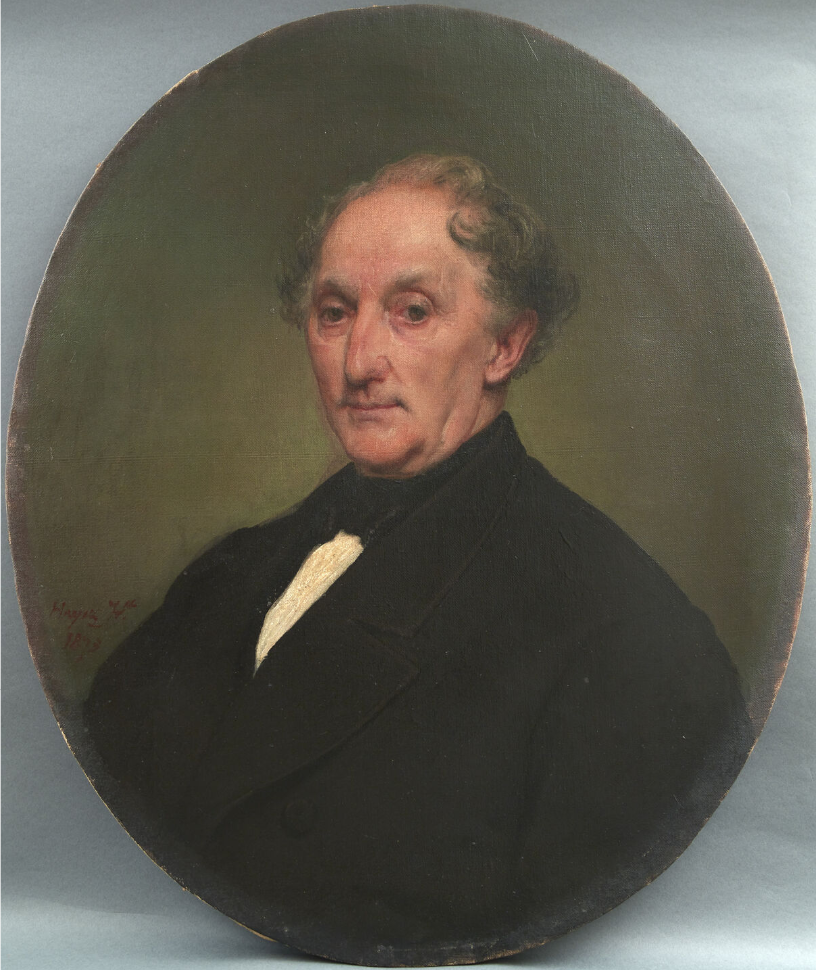This detailed painting portrays an elderly Caucasian man seated indoors, depicted from the abdomen up. The artwork is created in a cameo style against a rectangular canvas with slate gray corners. The focal point is an oval portrait with a smoky brown taupe background. The man, slightly balding, has receding, wavy hair that's gray on top and darker at the bottom, curling to the top of his ears. His complexion is light with a hint of redness on his nose and cheeks, and adorned with wrinkles and a few spots. 

The subject's dark brown eyes stare downward rather than meeting the viewer directly. He has a long, somewhat hooked nose, large eyes, a small mouth with pinkish lips, and a narrow face with a prominent chin. His right ear is partly obscured, while his left ear is fully visible. His eyebrows are bushy, and there's a slight mustache present.

For attire, he wears a period-appropriate black jacket with large lapels and a white shirt underneath, along with a black tie. The jacket is somewhat unkempt. The man's head appears small compared to his broad shoulders and chest. Enclosing the oval portrait is a greenish background with subtle shadows at the bottom. Near his right shoulder, there is some small, illegible writing. Overall, the portrait exudes a sense of history, perhaps dating back to the 19th or early 20th century.